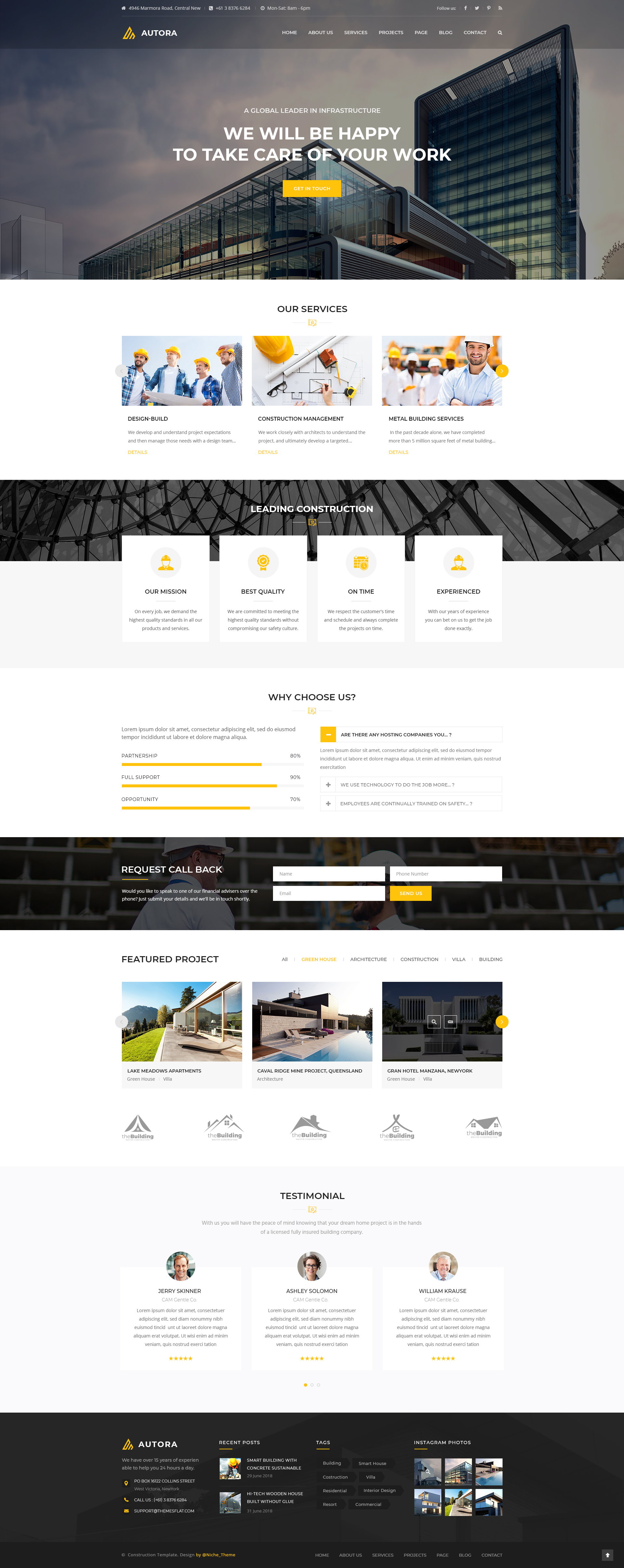The screenshot captures a comprehensive view of a company's website, seamlessly blending modern design elements with detailed content. At the top, the website displays its name accompanied by a small logo and a navigation menu. A striking grayscale background photo features a sleek glass building against the sky, highlighting the company’s architectural prowess.

Following the header, a prominent white section titled "Our Services" features three tiles, each with descriptive text outlining the various services the company offers. Beneath this, a gray and white section delves into the company's background and outlines the types of construction projects they undertake.

Next, a dedicated white area labeled "Why Choose Us?" lists compelling reasons to select this company over its competitors. This is followed by a black section inviting users to "Request Callback," where they can fill out their information to receive a follow-up. 

Further down, a "Featured Projects" section showcases the company’s active projects, alongside customer testimonials attesting to their quality and service. The webpage concludes with a typical footer, replete with links to significant pages and sections of the website, providing an easy-to-navigate user experience.